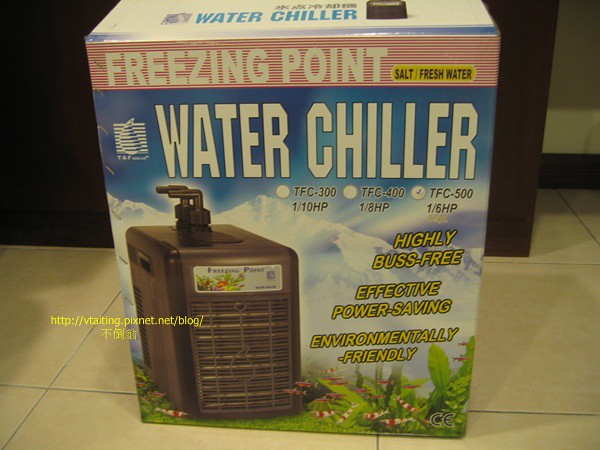The image showcases the front of a water chiller box, prominently featuring the text "Freezing Point Salt/Fresh Water" at the top amidst a design of red and white vertical lines. Just below this, "Water Chiller" is displayed in bold white text against a blue sky backdrop that transitions into snowy mountains and further down into a lush grassy meadow. The central part of the box contains an image of the black water chiller unit situated in a grassy area with surrounding bushes and small fish, an unusual combination given the mountainous background.

Beneath the "Water Chiller" heading are three bullet points detailing different models and their horsepower ratings: 
- TFC 300 1/10 HP (unchecked)
- TFC 400 1/8 HP (unchecked)
- TFC 500 1/6 HP (checked)

Highlighted in yellow text over the scenic imagery are the attributes "Highly Bus-Free, Effective Power-Saving, Environmentally Friendly." The top of the box is predominantly white with "Water Chiller" written in blue, accompanied by a small black square next to the word "Chiller." The bottom left corner of the box features a web address, "http://mytaking.pixnet.net/blog," followed by characters in a foreign language. The box is placed on light brown towels with gray grout visible between them, and in the background, there is a dark brown box.